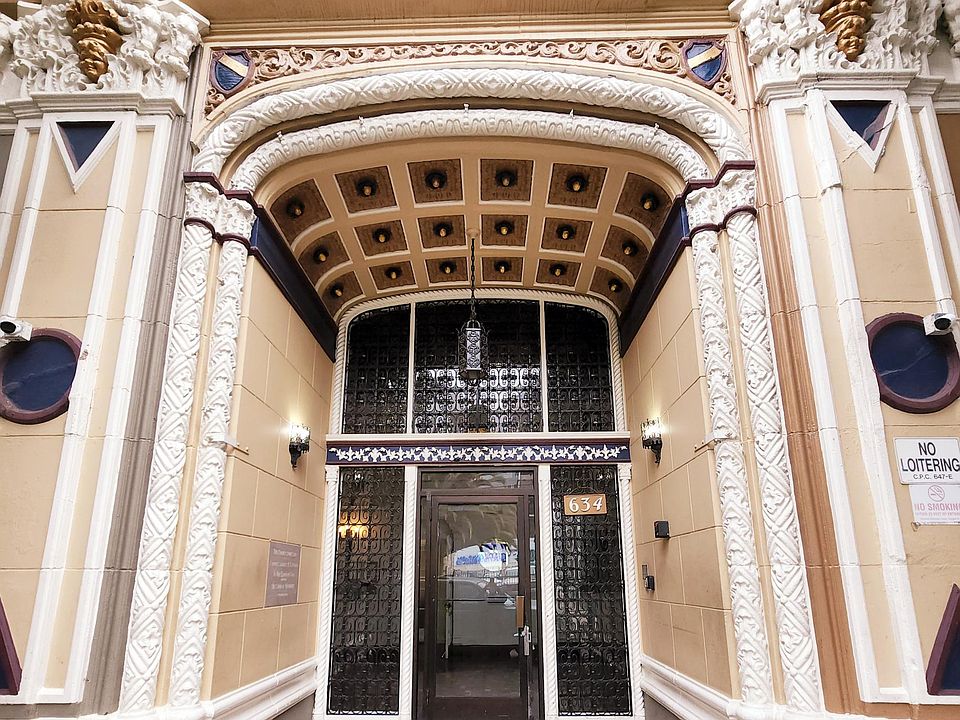The image depicts the front entrance of a grand, ornate building, showcasing a blend of intricate architectural details and modern surveillance elements. The facade is constructed from large beige blocks of stone, with a prominent entrance marked by the number 634. The entryway is framed by an arched opening that is more of a rounded rectangle, adorned with white sculpted pillars and decorative elements. Above the black wrought-iron and glass door is a ceiling divided into squares, each possibly housing a light fixture.

The entry pathway is lined with pinkish-beige tiles leading up to the door, which is surrounded by a see-through grate. The arches and surrounding walls feature elaborate white etchings with gold and navy blue accents, including glass-like blue circles that contain cameras. The building also has numerous surveillance cameras and lamps affixed to the exterior. Prominent signage warns against loitering (CPC 647-E) and smoking, emphasizing its strict policies. This scene is bathed in bright sunlight, highlighting the building's historical architectural style amidst modern functional elements.